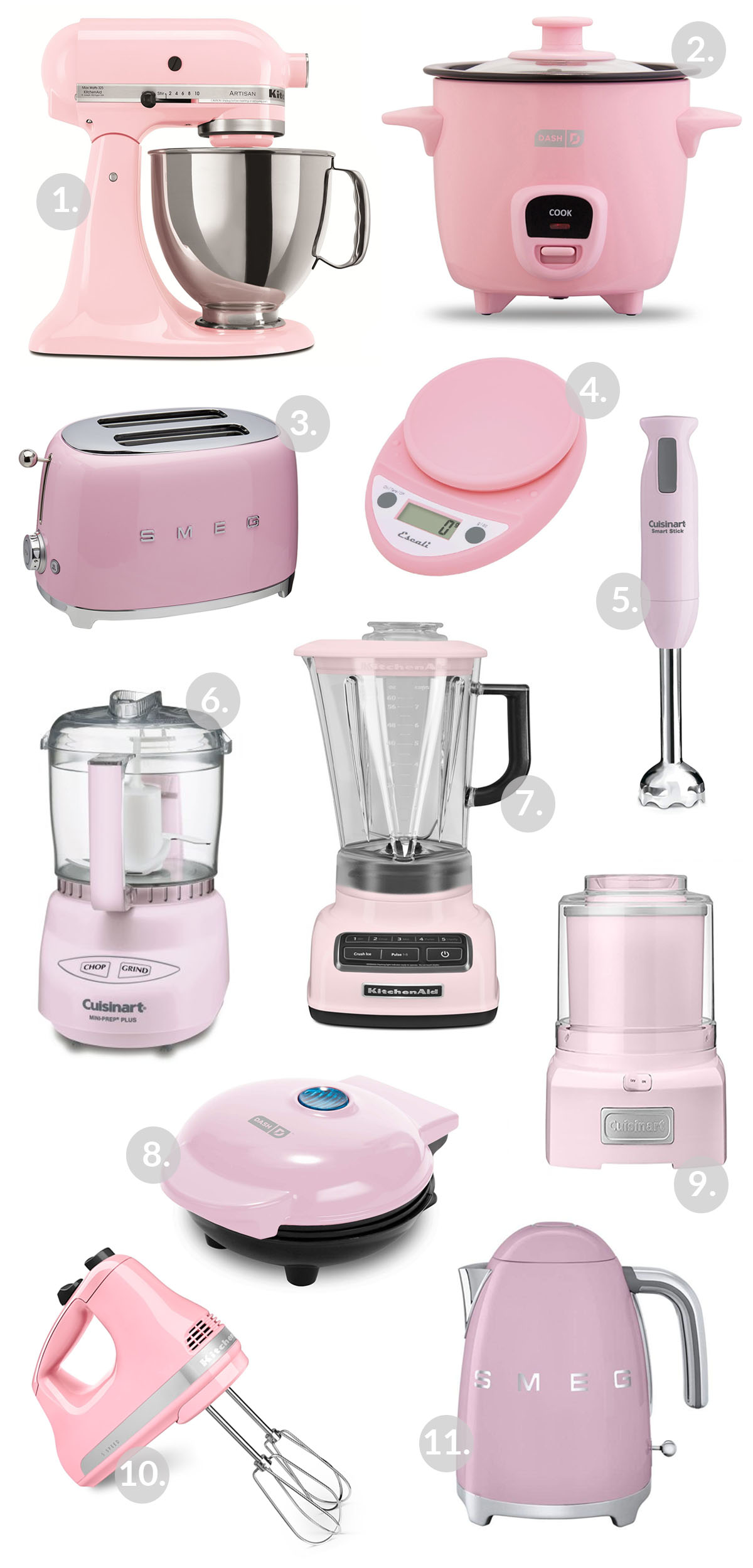This color photograph features a series of 11 numbered countertop appliances arranged against a white background, emphasizing a cohesive pink theme with stainless steel accents. At the top left, a stainless steel-bowled, pink KitchenAid mixer is prominently displayed. To its right, a pink crock pot with a black top and digital control panel sits. Below, from left to right, a chrome-topped pink toaster and a digital kitchen scale follow in sequence. Moving further right, a handheld pink mixer with a stainless steel attachment can be seen. On the next row, from left, a Cuisinart food processor with a clear plastic top and pink base with a handle is followed by a blender boasting a clear container and matching pink base and lid. 

In the row below, a pink countertop griddle or waffle maker, featuring a black base and a pink lid, is visible. Adjacent is a pink appliance resembling an ice cream maker or juicer with a clear top. Finally, in the bottom row, a pink hand mixer with two stainless steel attachments is positioned on the left, next to what appears to be a pink coffee or tea brewer with a stainless steel handle and pouring spout, possibly labeled with the brand name SMEG. The entire collection is meticulously displayed in five rows, each appliance consistently featuring pink aspects in their design, marked by white-numbered gray circles from 1 to 11 for easy identification.